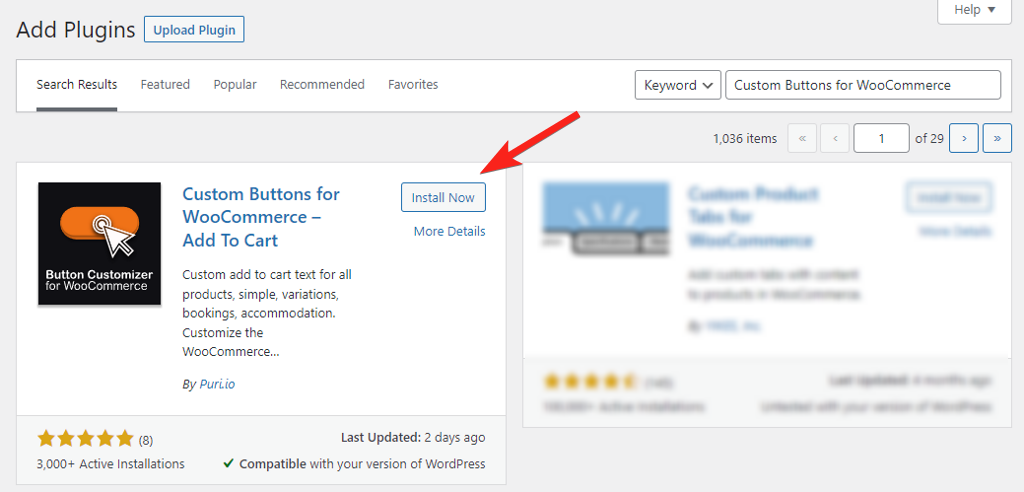The image features a gray background with the text "Add Plugins" written in black. Dominating the top section, there's a blue-outlined banner with the text "Upload Plugin" in blue against a white background. On the right, a white banner contains the word "Help" with a downward-pointing black arrow. 

Below this, another white banner runs horizontally displaying various categories: "Search Results," "Featured," "Popular," "Recommended," and "Favorites." The "Search Results" category is underlined in dark gray, highlighting it as the active selection. 

On the right side, two dropdown menus are present: the first one labeled "Keyword" with a downward arrow, and the second one featuring text about custom buttons for WooCommerce.

A prominent feature is a red arrow pointing to a section on the left, which highlights a plugin titled "Custom Buttons for WooCommerce - Add to Cart" in blue. This section features a blue-outlined button that says "Install Now," which is also the focus of the red arrow. Below this button, there’s another blue link that says "More Details." 

Further down, there is text describing the plugin's features: "Custom add to cart text for all products, simple variations, bookings, accommodation," followed by the word "WooCommerce." The word "Buy" is also present followed by "Pureleo" in blue. This plugin boasts a rating of five gold stars from 8 reviews, over 3,000 active installations, and was last updated two days ago. It is marked as compatible with the user's version of WordPress. 

The plugin's logo, a black box with an orange banner and two white circles with a white arrow pointing to it, accompanies the description. It also states "Button Customizer for WooCommerce." 

To the right side, a muted box is present, making it difficult to discern its contents, although stars are visible. Above this, a small notation reads "1,036 items" with an arrow pointing, and a label stating "Number 1 of 29."

This detailed layout provides a comprehensive overview of the current plugin being viewed and its essential details.